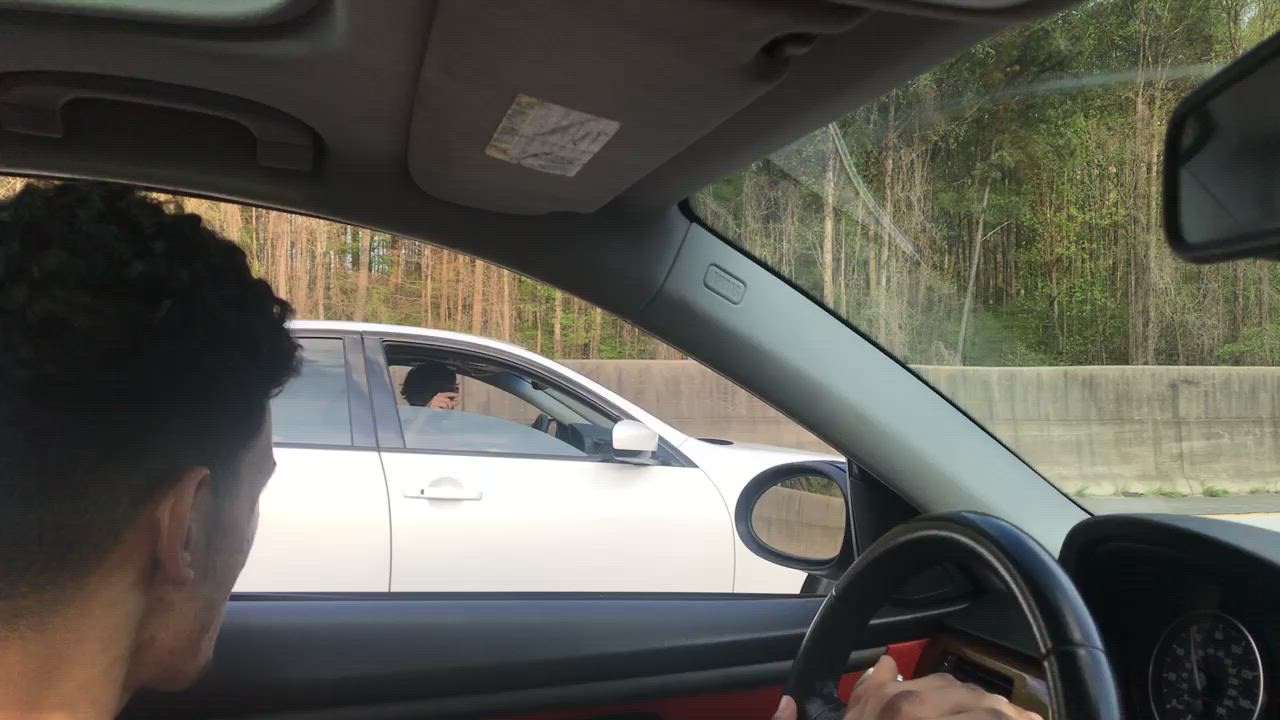This is a color photograph taken from inside a car, with the perspective focused through the driver's side window. Inside the car, the driver, a young man with dark hair, has his hands on the steering wheel and is gazing sharply to his left. The car's interior includes light gray upholstery with a brownish-red strip on the door. Outside, to the left of the car, there is a white car with its passenger side window partially rolled down. The person inside the white car appears to be making a gesture with their hand, seemingly engaged in conversation or interaction with the driver in the foreground. The background features a stone wall about three to four feet tall, separating the road from a densely treed area with thin trunks and abundant green foliage. The scene conveys a moment of possible frustration or communication between the two drivers on a highway.